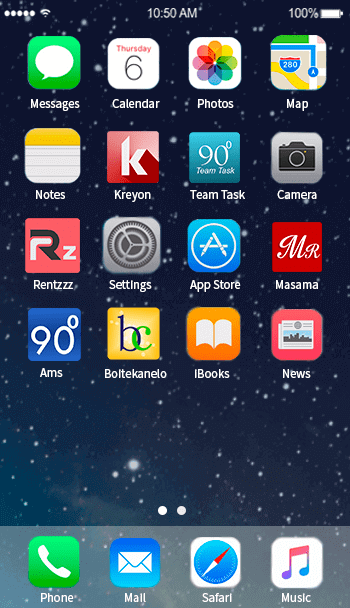This screenshot captures the home screen of an iPhone at 10:50 AM, with the battery fully charged at 100%. The lineup of apps is diverse, featuring both standard iPhone applications and some lesser-known, possibly custom apps. 

In detail, the home screen includes the following apps:
- **Messages**: The familiar green speech bubble icon for texting.
- **Calendar**: Displaying the date "Thursday the 6th."
- **Photos**: The colorful flower icon.
- **Maps**: Represented by the Apple Maps icon.
- **Notes**: The yellow notepad icon.
- **Crayon**: A red icon with a 'K', likely a specialized app.
- **Team Task**: Featuring a "90" on the icon, indicating task management or productivity tracking.
- **Camera**: The standard camera icon.
- **Rentszzz**: An app with three Z's, purpose unclear.
- **Settings**: The traditional gears icon.
- **App Store**: The blue "A" icon.
- **My Asthma**: An app associated with a song by Ghost, though the exact nature of the app is unclear.
- **iBooks**: The standard book icon.
- **News**: Displaying the typical news icon.

On the bottom bar of the home screen, the frequently used apps include:
- **Phone**: The green handset icon.
- **Mail**: The envelope icon.
- **Safari**: The compass icon for web browsing.
- **Music**: Represented by the musical note icon.

The background shows a mix of standard iPhone apps and unique custom apps, which may be experimental or not widely released.